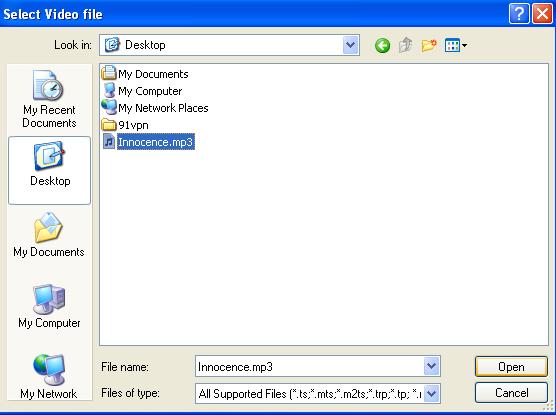The image depicts a classic Windows XP file selection window from the early 2000s, characterized by its blue banner with white text at the top reading "Select Video File." At the top right, there is a small blue question mark icon and a red "X" for closing the window. Below the banner, a dropdown labeled "Look in" is set to the "Desktop."

On the left side of the window, there's a navigation pane listing several locations: "My Recent Documents," "Desktop," "My Documents," "My Computer," and "My Network." The "Desktop" option is selected and displays a list of items in the main window area. These items include: "My Documents," "My Computer," "My Network Places," "91 VPN," and "innocence.mp3," with "innocence.mp3" being highlighted, indicating it is about to be opened. 

On the right side of the window, several icons represent various functions. At the bottom of the pane, there's a drop-down menu for "Files of type" currently set to "All Supported Files," and the "Open" button is highlighted, with a "Cancel" button next to it.